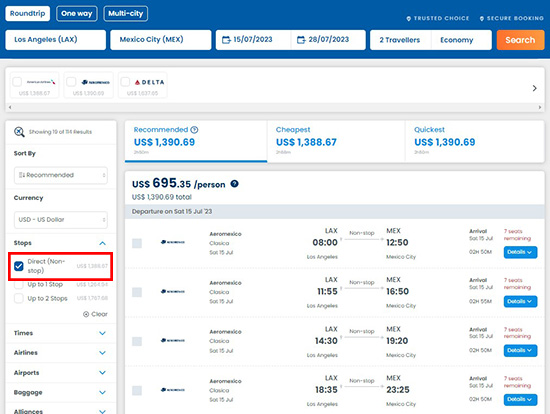A detailed screenshot of flight information is presented, illustrating travel details for a journey from Los Angeles to Mexico City. The top left corner of the screenshot features options for different types of trips: roundtrip, one-way, and multi-city. The flight dates are specified as July 15, 2023, to July 28, 2023, accommodating two economy-class travelers.

On the left side of the image, a filter section is visible, with a red rectangle outlining the button labeled "Direct, Non-stop." On the right side, several pricing options are displayed: the recommended flight costs $1,390.69, the cheapest available is priced at $1,388.67, and the quickest option is also $1,390.69, breaking down to $695.35 per person. Additionally, detailed flight information, including arrival and departure times, is shown.